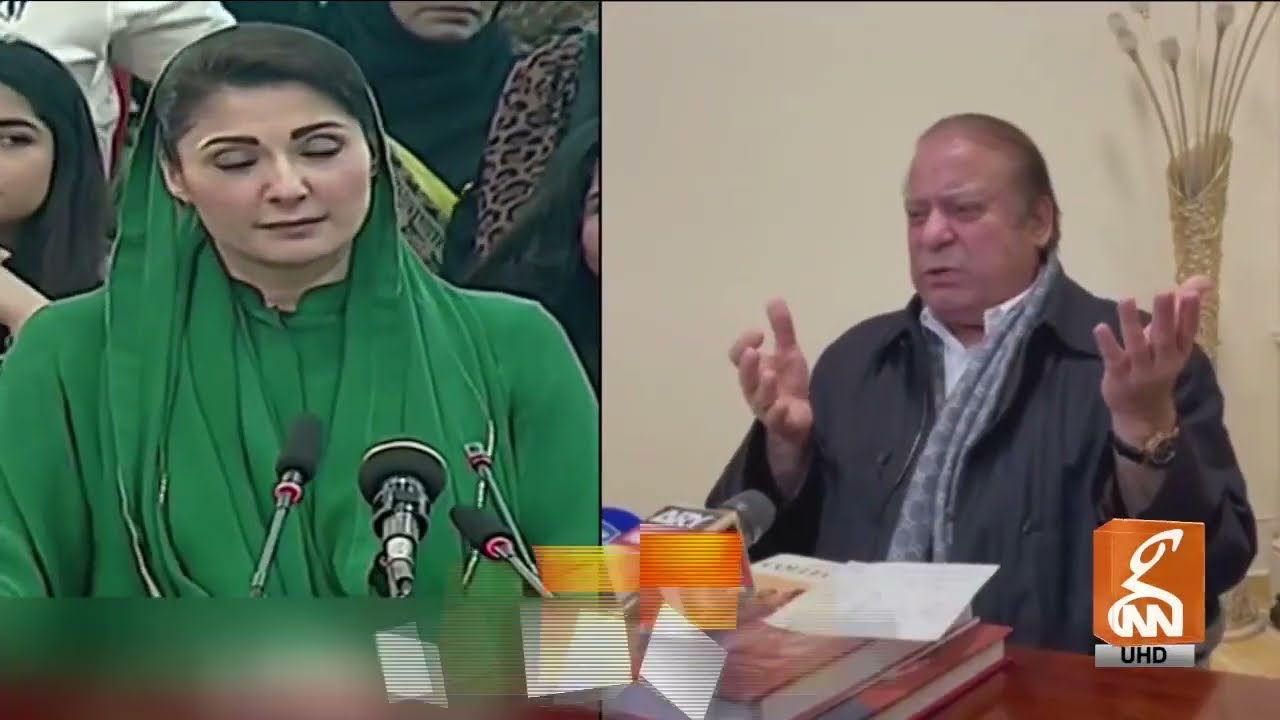In this image, two distinct photographs are side-by-side, each showcasing different individuals and settings. On the left side, a woman dressed in a green outfit, which includes a headscarf, stands before multiple microphones with her eyes closed. She is framed by the faces of several other women positioned behind her, hinting at a public event or gathering. On the right side, a man is seated indoors at a table that holds several books and a microphone. He is dressed in a black coat, possibly a windbreaker, with a gray scarf and a white shirt with a popped collar. His expression appears intense, with furrowed eyebrows and a speaking posture, suggesting he might be responding to or addressing the situation involving the woman. Both settings are rich in color, featuring browns, tans, greens, reds, oranges, and more. At the bottom right corner of the composite image, there is a logo in white and orange with the text “UHD,” indicating a possible broadcast or channel identifier.